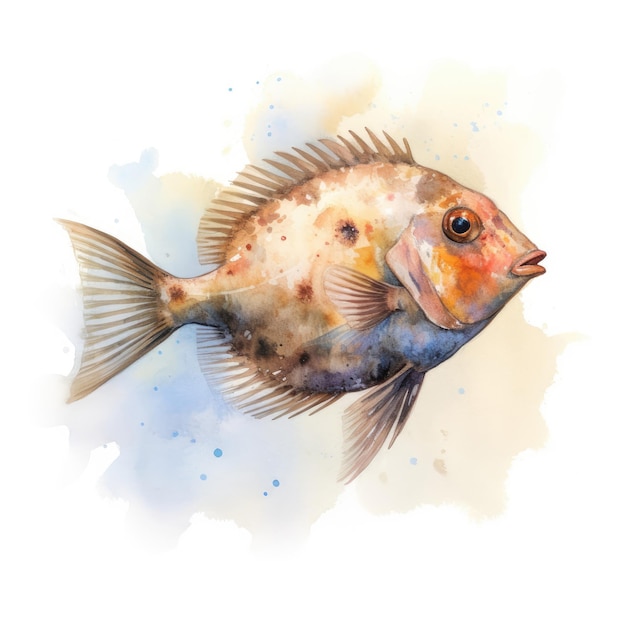This image depicts a detailed watercolor illustration of a fish, rendered in a style that is both artistic and realistic. The fish, presented on a white background, is surrounded by soft, faded splashes of blue and orange, creating a watery, bleeding effect. The fish itself exhibits a variety of colors and intricate details: its body transitions from a pale yellow to a reddish-orange towards the face, which has a rosy hue and pink lips. The eye is large and bulbous with a dark brown iris and a black pupil. The underbelly of the fish features hues of blue and purple, while the top part is primarily white with light brown and dark brown speckled markings.

The fish's scales are described as dark brown and translucent, adding to the detailed texture of the illustration. Its dorsal and tail fins are serrated and spiky, while the fins near its gills and under its face are smoother. The overall shape of the fish is almond-like, and it is depicted from a side view, swimming to the right with an open mouth. The background enhances the fish’s vibrant colors with light blue and tannish translucent spots, emphasizing the watercolor technique used in the painting. This piece combines soft and gentle watercolors with sharper, more vibrant tones, making it a visually engaging and detailed work of art.